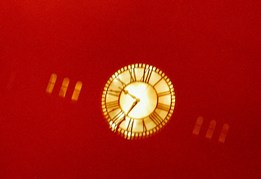The image features a prominently lit, shiny gold clock with Roman numerals, displaying the time as approximately 9:35. The clock, round in shape, occupies a very small portion at the center of the frame. The background is a muddy red, casting a surreal and somewhat misty glow across the scene. This red backdrop gives the clock a contrasting appearance, making it stand out vividly. Surrounding the clock are six thin, vertically oriented gold bars or narrow windows, three on each side, which are more distinct on the left. These bars add symmetry and a decorative touch to the simple yet striking image. The clock's hands, fashioned in an arrow-point style, and the Roman numerals rendered in a brownie red color, enhance the classic aesthetic of the clock face. The top-left of the image is slightly illuminated, suggesting a light source outside the frame, which further accentuates the glowing golden color of the clock.